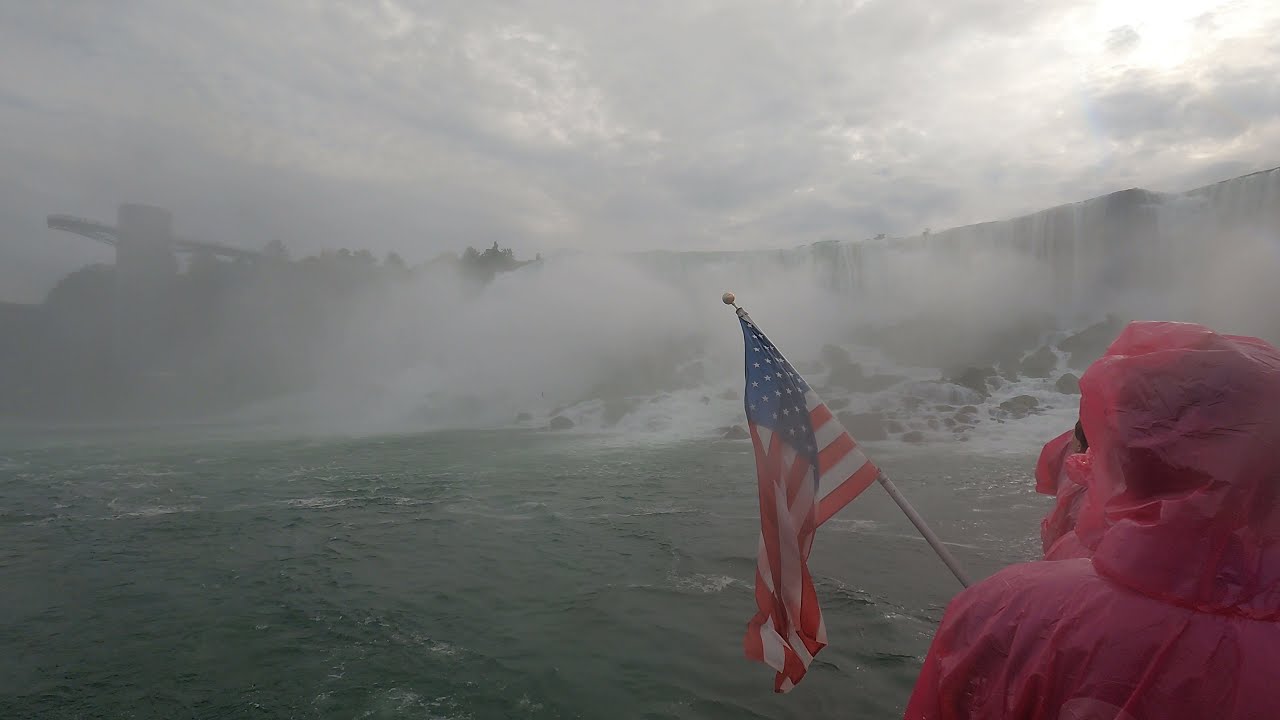This image depicts a cloudy, overcast day at Niagara Falls, with a striking waterfall creating a massive mist in the background. Central to the image is the powerful cascade of water crashing down, surrounded by a hazy atmosphere that gives the scene a grainy, dream-like quality. The water below appears choppy and greenish, likely from the turbulence of the falls. In the lower right corner stands a person wearing a pink or red plastic raincoat, typical of those worn by visitors to shield themselves from the spray. This individual is holding an American flag tilted at an angle of about 60 degrees. Their presence adds a touch of color and a sense of scale to the majestic scene. To the left of the falls, there is a structure, possibly an overlook building, hinting at the human interaction with this natural wonder. The image's dominant colors are the pink and red of the raincoat, the red, white, and blue of the flag, and the greenish hues of the water, all under a sky filled with light gray clouds. A hint of sunlight bursts through the clouds on the top right, adding a subtle, ethereal light to the otherwise gray-toned image.